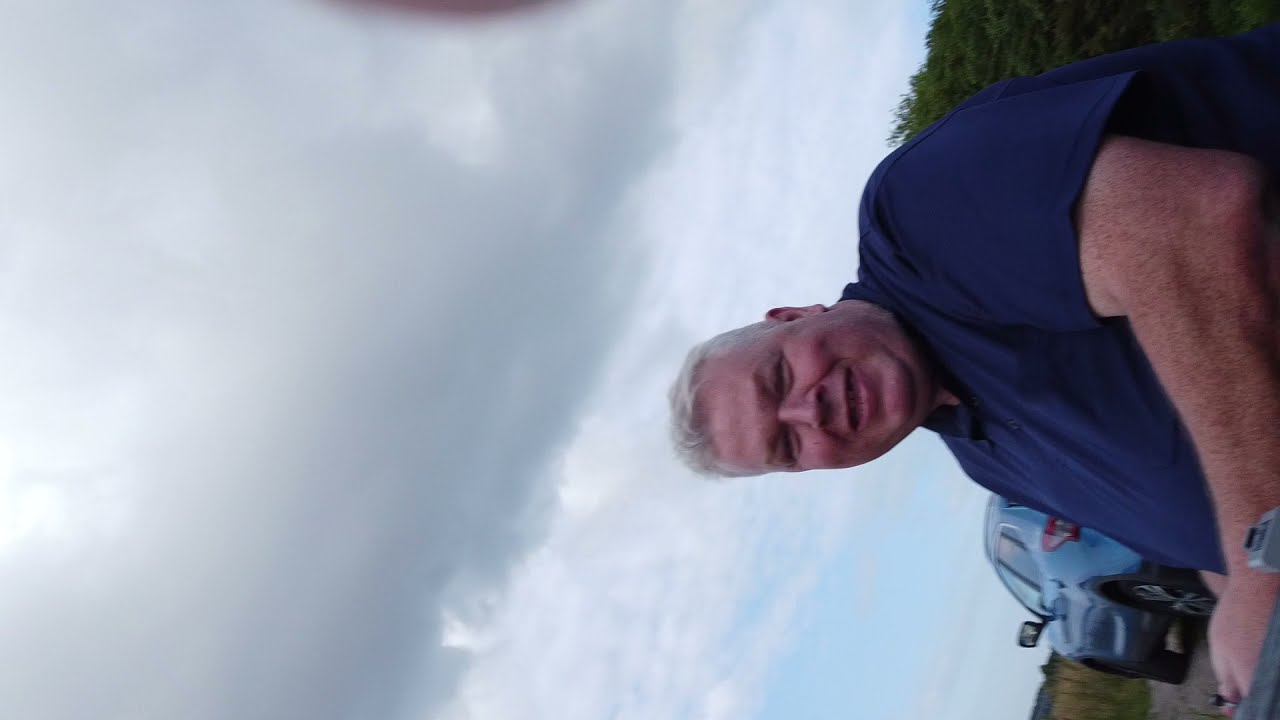In this sideways photograph, we see an older Caucasian man standing on the right side of the image. He has short gray hair and is smiling slightly while wearing a dark blue polo shirt. The man appears to be heavyset and is positioned in front of a light blue SUV that is parked on a road. Behind him, there are visible trees and greenery. The sky above is filled with thick, flat clouds, some of which are dark and saturated with water, creating a gloomy atmosphere.